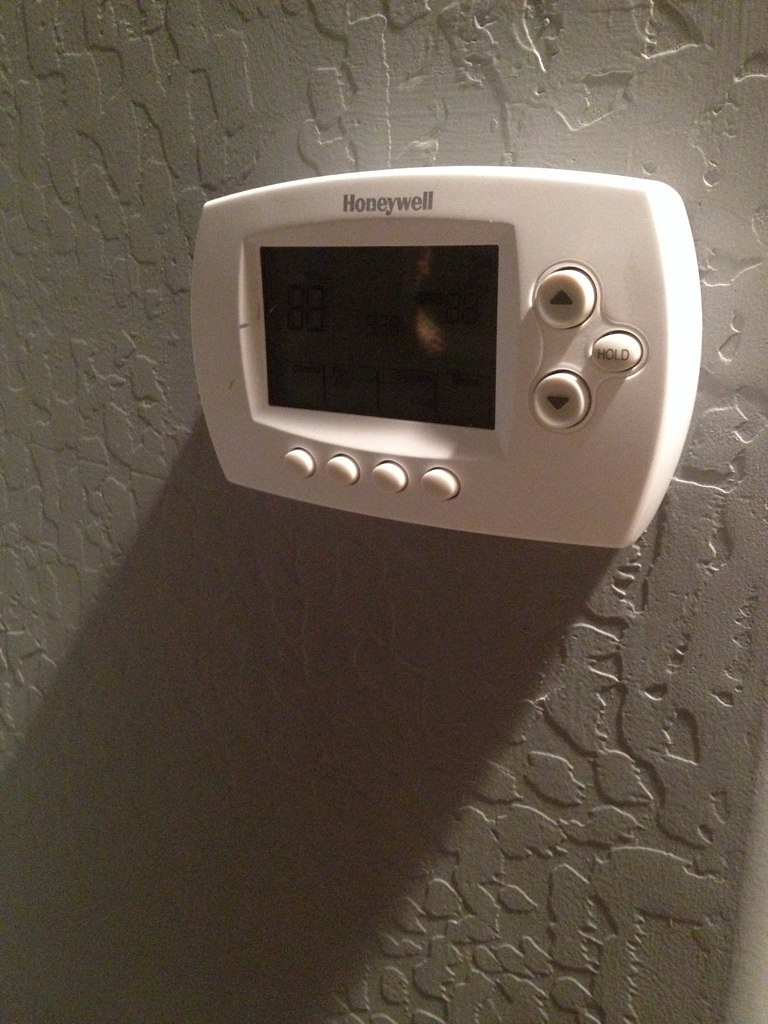This photograph showcases a Honeywell thermostat mounted on a textured white wall. The wall's texture is subtly visible, providing a tactile background to the thermostat. Positioned about two-thirds up the image, the white thermostat features a rectangular shape with gently rounded sides. The screen at the center of the device appears very dark and unreadable, suggesting that it may be turned off or inactive. Above the screen, the Honeywell brand name is displayed.

Below the screen, there are four white rectangular buttons, while to the right of the screen, three additional buttons are placed vertically: an up button, a down button, and a "hold" button. The device looks like a model that might be around 10 years old, implying it is neither very recent nor too outdated.

A light source from above illuminates the scene, casting a distinct shadow of the thermostat downwards towards the bottom left corner of the photograph. On closer inspection, the screen seems to faintly outline the digits "88," though it is unclear if this display is accurate or just an illusion. Overall, the image captures a well-used Honeywell thermostat against a detailed white wall, accompanied by subtle lighting and shadows.